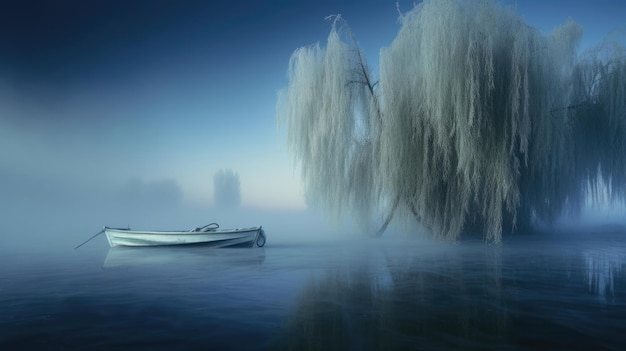The image depicts a serene, possibly edited or painted winter scene of a small, white rowboat floating in the center of a crystal-clear, blue lake. The boat, which has a tan top or wooden interior, sits anchored in place with a rope extending from its left side into the water. At the front of the boat, a fishing net is faintly visible. To the right of the boat, a large, majestic willow tree stands, its branches seemingly covered in white, resembling frosted icicles or heavy snow, giving the impression of a frozen moment. The background is shrouded in a delicate haze or fog, revealing faint shadows and rock formations along with some barely visible trees on the shoreline to the left. This ethereal scene, with its harmonious palette of blue and white, has no text to distract from its peaceful, wintery ambiance.